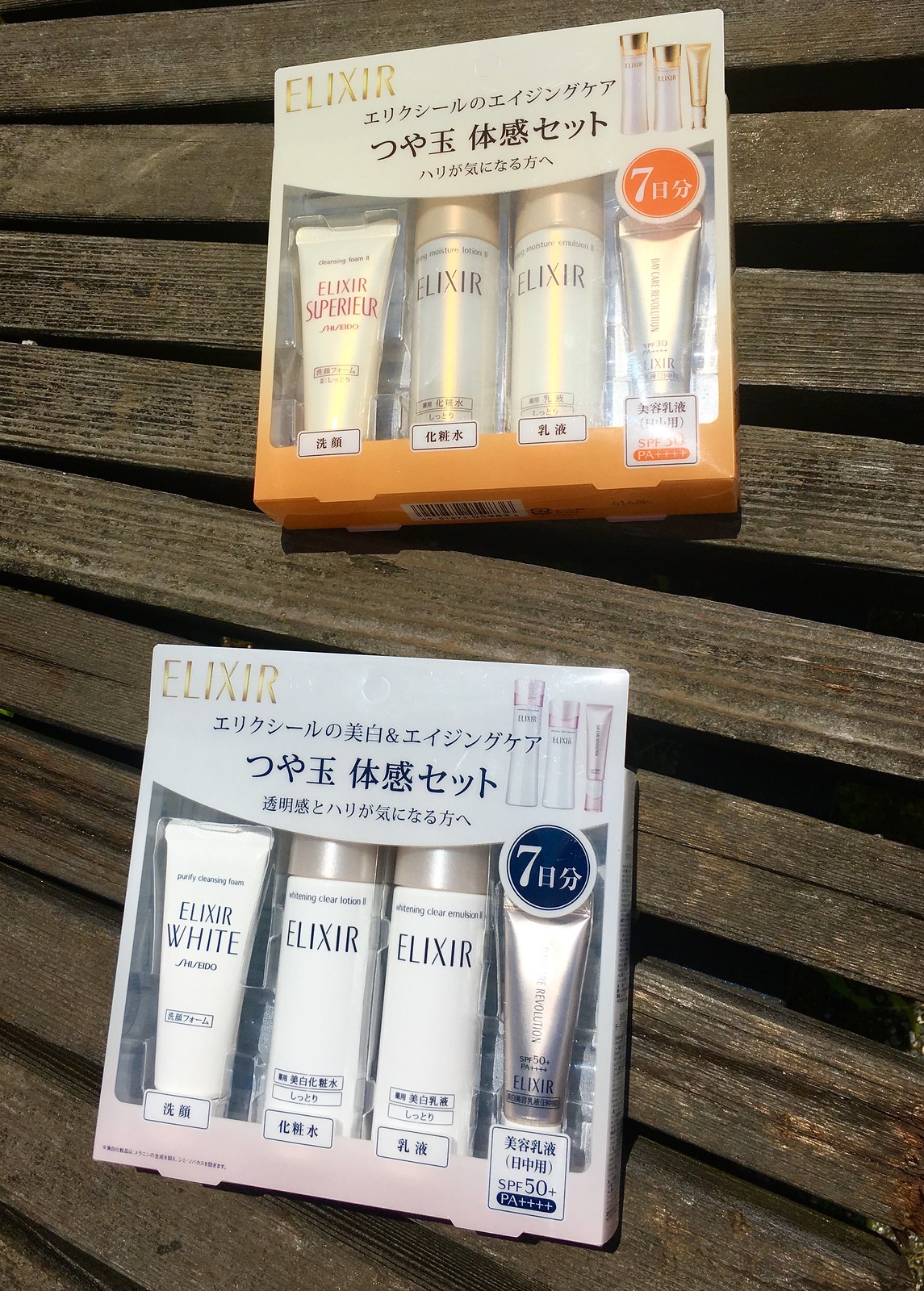The image displays two women's beauty products resting on a dark brown wooden surface composed of evenly spaced slats, allowing glimpses of a black background through the gaps. Both products appear to be from the same brand as indicated by the word "Elixir" at the top of each package, although the rest of the labeling is in either Japanese or Chinese. 

The package on the top is predominantly white with orange trim and holds four distinct bottles inside, each featuring slight variations. The bottle on the left is labeled "Elixir White," the two in the middle simply say "Elixir," and the bottle on the right is somewhat blurry, only showing the word "Elixir" at the bottom. Despite the blurriness, an SPF 50+ icon is visible on the bottom part of the image, with the upper part suggesting either SPF 30 or 50, although reflections from sunlight obscure the details.

The second package, positioned below, mirrors the first in size and structure but is adorned with light purple trim instead of orange. It also contains four bottles with similar, yet distinct, appearances. Each package features a circular emblem marked with "7H" followed by what seems to be a number. On the top package, this emblem is orange, while on the bottom, it is blue.